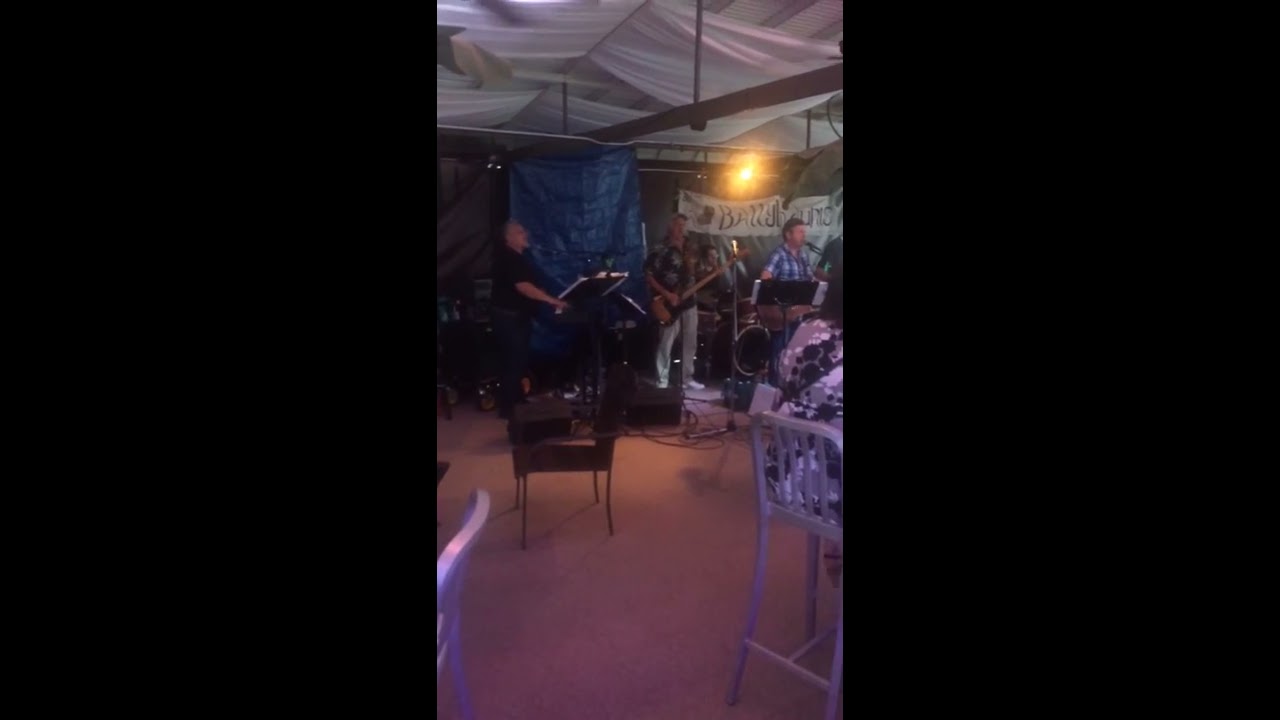The image captures a frame from a vertical video of a band performing at what appears to be a wedding venue, possibly at Memphis Pavilion. This makeshift setup is characterized by a tent-like white cloth ceiling and a light-colored floor. Scattered around the floor are random chairs, including black, white, and silver ones, and stools, with one visibly occupied by an attendee in a lavender and dark blue printed top. The band consists of two or three vocalists, with one playing the piano and another on guitar, along with a bassist and a drummer in the background. 

One band member is dressed in a black top and dark bottoms, another in a black printed top with light-colored trousers while playing guitar, and a third sporting a blue plaid top, possibly the lead singer as there's a microphone in front of him. Despite the low lighting that makes the image appear underexposed and dark, a single yellow light illuminates the band. Overhead, draped fabrics or white cloths hang, contributing to the venue's ad hoc decor. A crumpled, unreadable banner hangs in the back, framed by blue and black cloths. In the foreground and to the left, a couple of figures are partially visible, adding to the candid and personal ambiance of this indoor, low-key celebration.